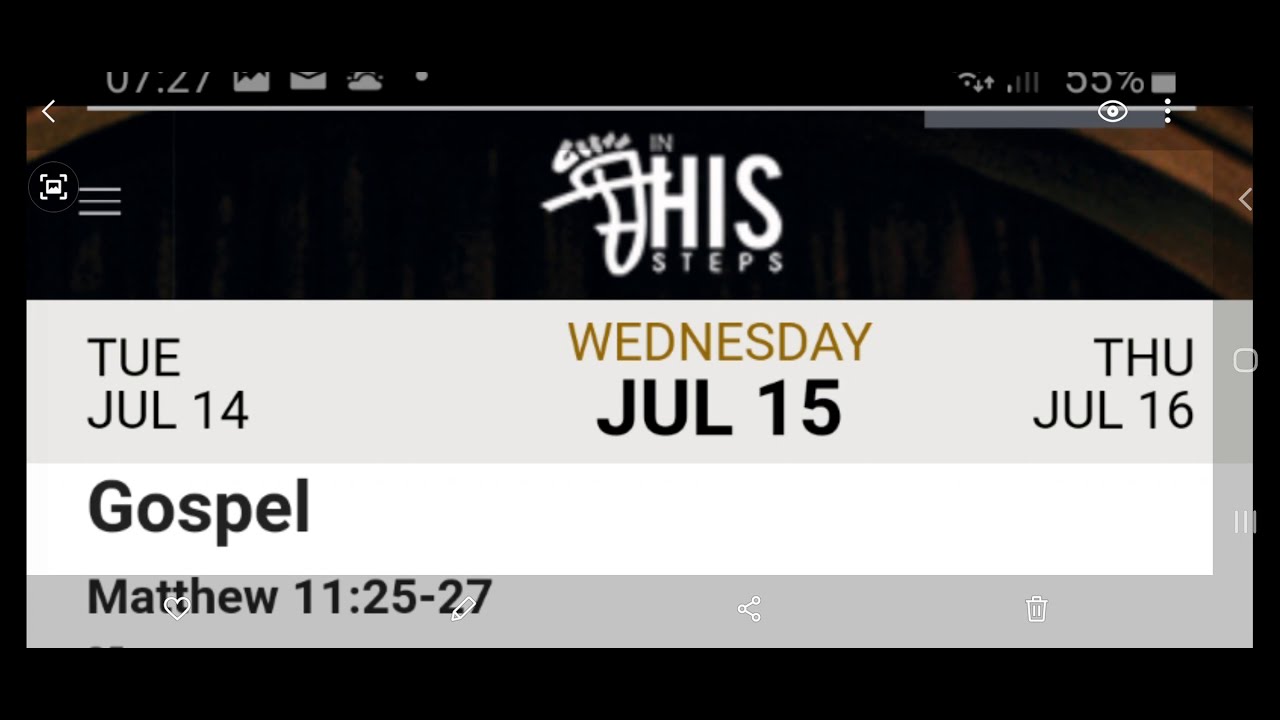The image is a landscape-oriented screenshot taken from a phone, characterized by a plain black background. At the very top left, the partially visible time shows 7:27, accompanied by icons such as a mail logo, an envelope, and a cloud. On the top right, the battery is at 55%, with two active signal bars also partially cropped out. The main content in the center features a caption with the text "In His Steps," where "His" is prominently displayed in a large bold white font, while "In" and "Steps" are smaller. Below this, a calendar layout presents three dates: "Tuesday, July 14th," "Wednesday, July 15th," and "Thursday, July 16th," all in black font on an off-white background. "Wednesday, July 15th" is highlighted in a gold color. Under these dates, the text reads "Gospel, Matthew 11:25-27" in black font. The entire calendar layout is framed by a thin black border.